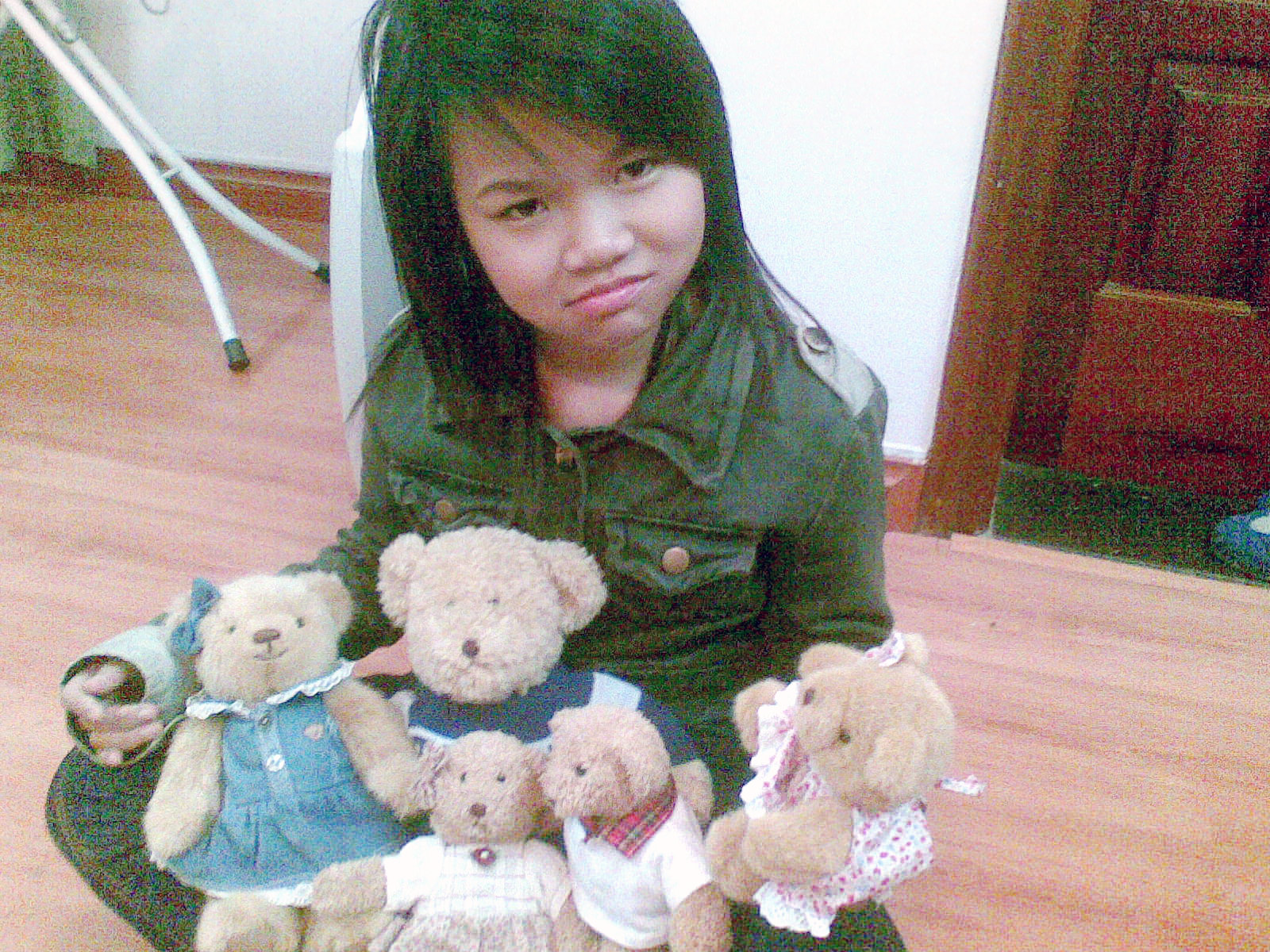In this blurry, out-of-focus photograph, a young Asian girl with brown hair and typical Asian features is sitting cross-legged on a brown hardwood floor. She is wearing a button-up denim jumpsuit adorned with many small buttons, a collar, and shoulder straps. The girl is looking up at the camera with a frown, her expression almost one of disgust. Nestled in her lap are five teddy bears of various sizes, seemingly representing a family: the dad, mom, and three children. The teddy bears are dressed with the mom in a denim dress and bow, and the children in little white shirts. The background reveals a brown wooden door and the legs of an ironing board visible in the upper right corner. The image appears pixelated and seems to have a filter applied.